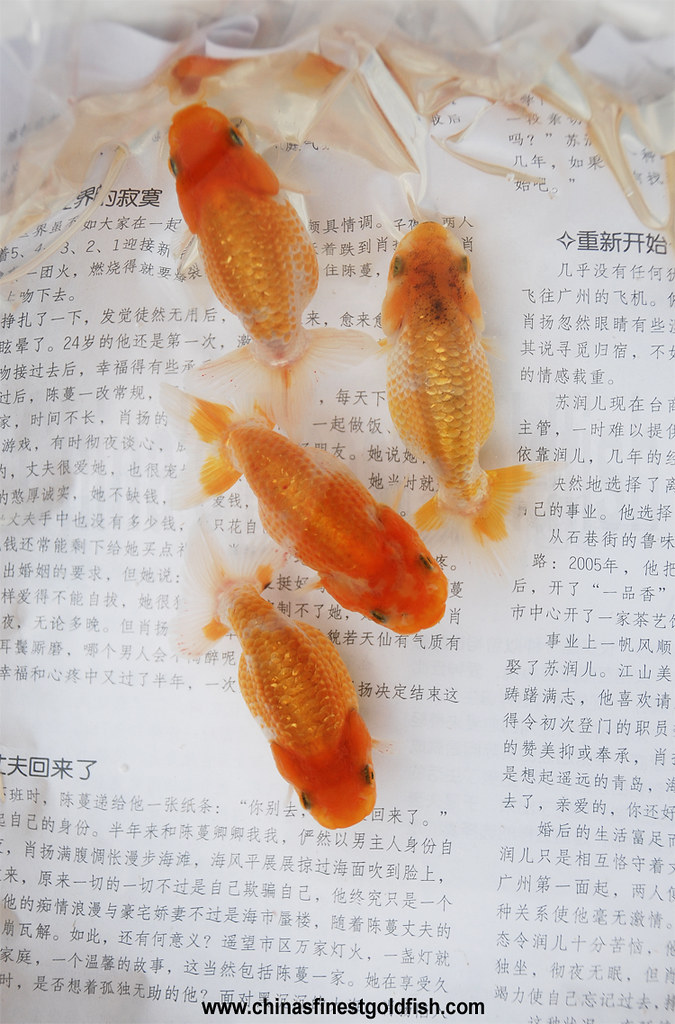This image showcases four plump goldfish with varying shades of vibrant orange scales and lighter fins, viewed from the top down. The goldfish, whose heads are the most intensely orange, are situated inside what appears to be a plastic bag, evident from the distinctive wrinkled reflections near the top of the image. The bag containing the fish is placed over a piece of paper or a book covered in Chinese characters. There's a watermark at the bottom center of the image that reads "www.chinasfinestgoldfish.com." The background text is completely in Chinese, contributing an element of cultural context to the setting.